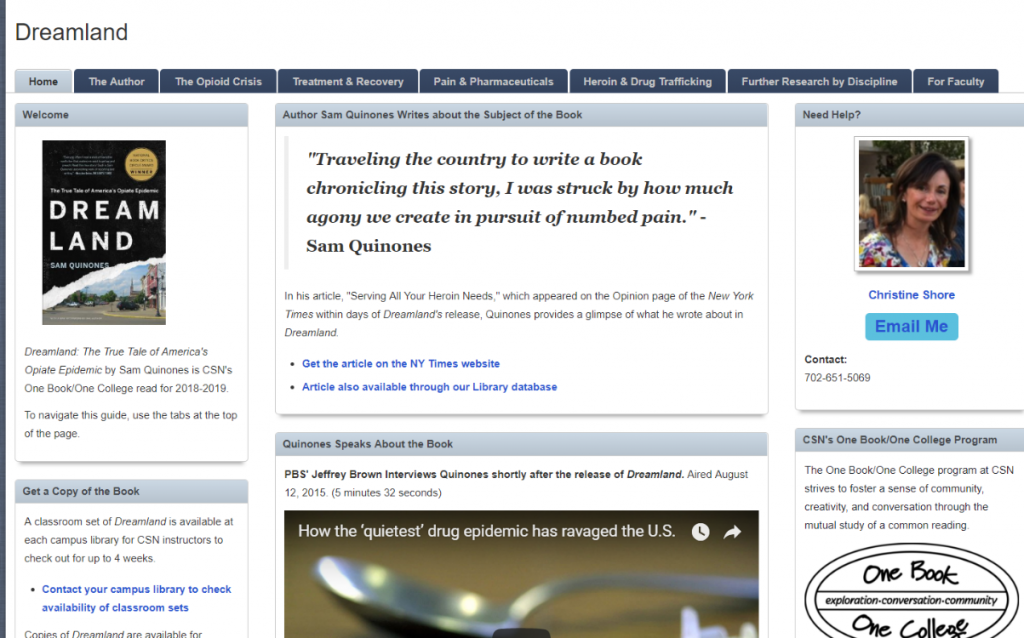This is an image of an author's homepage on CSN's website, centered around the book "Dreamland" by Sam Quinones, which is featured as the "One Book, One College" read for the 2018-2019 academic year. The website serves as a guide for navigating various resources related to the book.

**Description of the Page Layout and Features:**

1. **Top Left Corner:**
   - A label that reads "Dreamland by Sam Quinones."
   - The statement "Dreamland: The True Tale of America's Opiate Epidemic by Sam Quinones is CSN's One Book, One College Read for 2018-2019," which introduces the book and its significance.
   - Navigation tabs listed horizontally, including:
     - Home (currently selected and highlighted in gray with dark blue text)
     - The Author
     - The Opioid Crisis
     - Treatment and Recovery
     - Pain and Pharmaceuticals
     - Heroin and Drug Trafficking
     - For Research by Discipline
     - For Faculty

2. **Welcome Section:**
   - "Welcome" greeting along with an introduction to the page’s contents and purpose.
   - Instructions for using the guide, including obtaining a copy of the book.

3. **Middle of the Page:**
   - Extensive information about the book and the author.
   - A quote by Sam Quinones explaining his journey across the country while writing "Dreamland."
   - Mention of his article, "Serving All Your Heroin Needs," which appeared in the New York Times.

4. **Imagery and Multimedia:**
   - A picture of a middle-aged woman with long brown hair, wearing a floral top, identified as possibly Christine Shore, who offers assistance via an "Email Me" button and a contact number (702-651-5069).
   - A video of Sam Quinones being interviewed by PBS's Jeffrey Brown about "Dreamland," providing in-depth insights into the book.

5. **Right Sidebar:**
   - Contact information for Christine Shore.
   - Details about CSN's "One Book, One College" program, which aims to foster community, creativity, and conversation through a mutual study of the book.
   - The program's logo with the words "Exploration, Conversation, Community."

This detailed caption provides a thorough overview of the features and content found on the college's webpage dedicated to "Dreamland" by Sam Quinones.